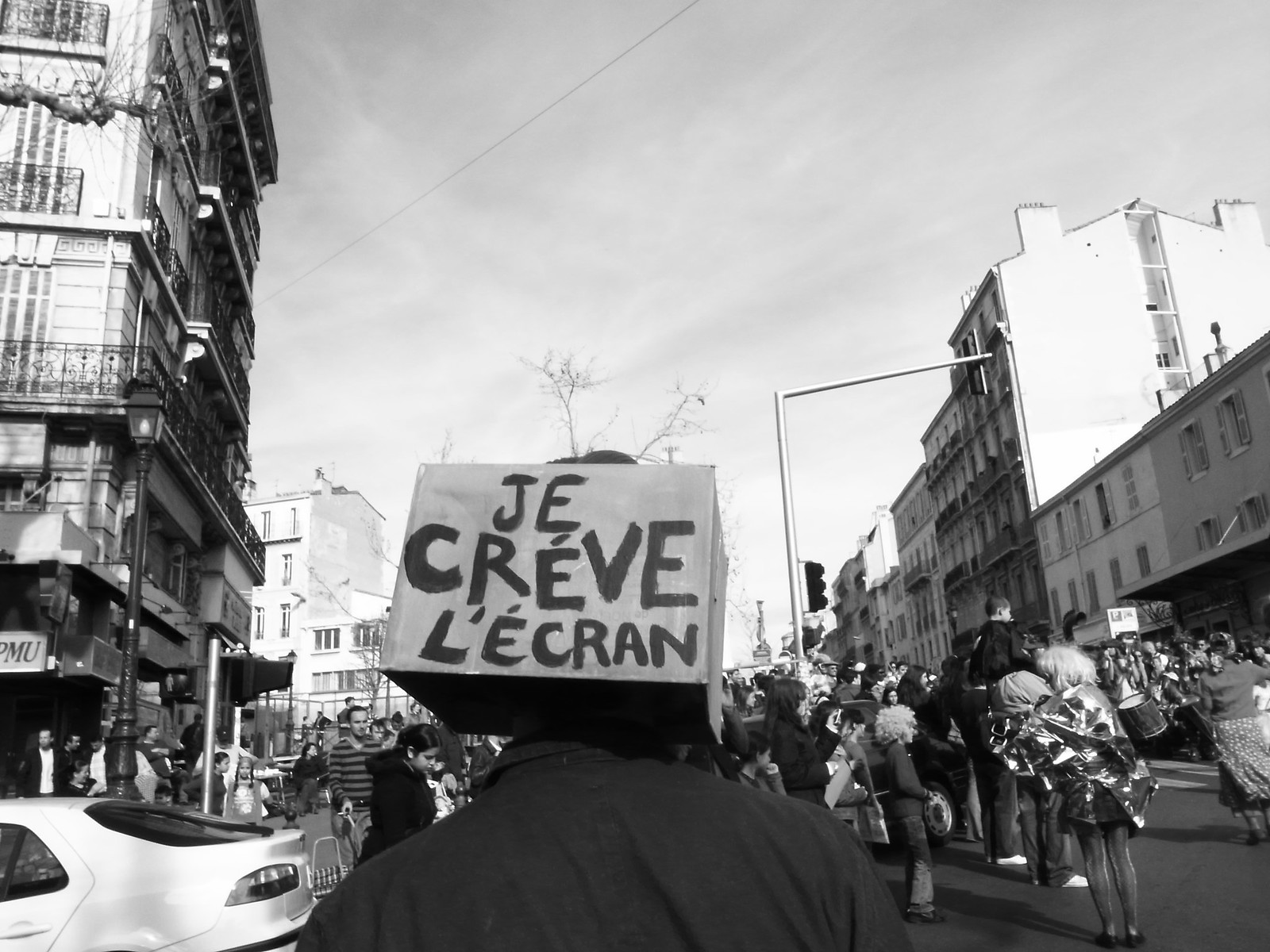The photograph, rendered in black and white, captures what appears to be a vintage scene, possibly from a protest or parade. Set amidst a cityscape, the image is flanked by tall buildings: to the left, a very old 5 or 6-story stone structure and to the right, a more modern 6-story edifice made of wood or brick. Dominating the foreground is a young man whose head is encased in a cubic, paper box with the text "J-E-C-R-E-V-E-L-E-C-R-A-N" written on it, suggesting a message in French. He's surrounded by a bustling street filled with people who are either walking or standing, some appearing to engage in activities typical of protest events, such as playing drums. The photograph, with clear skies above and a streetlamp positioned centrally, evokes a meticulously composed piece of street photography, capturing the essence of a public gathering in a bygone era.